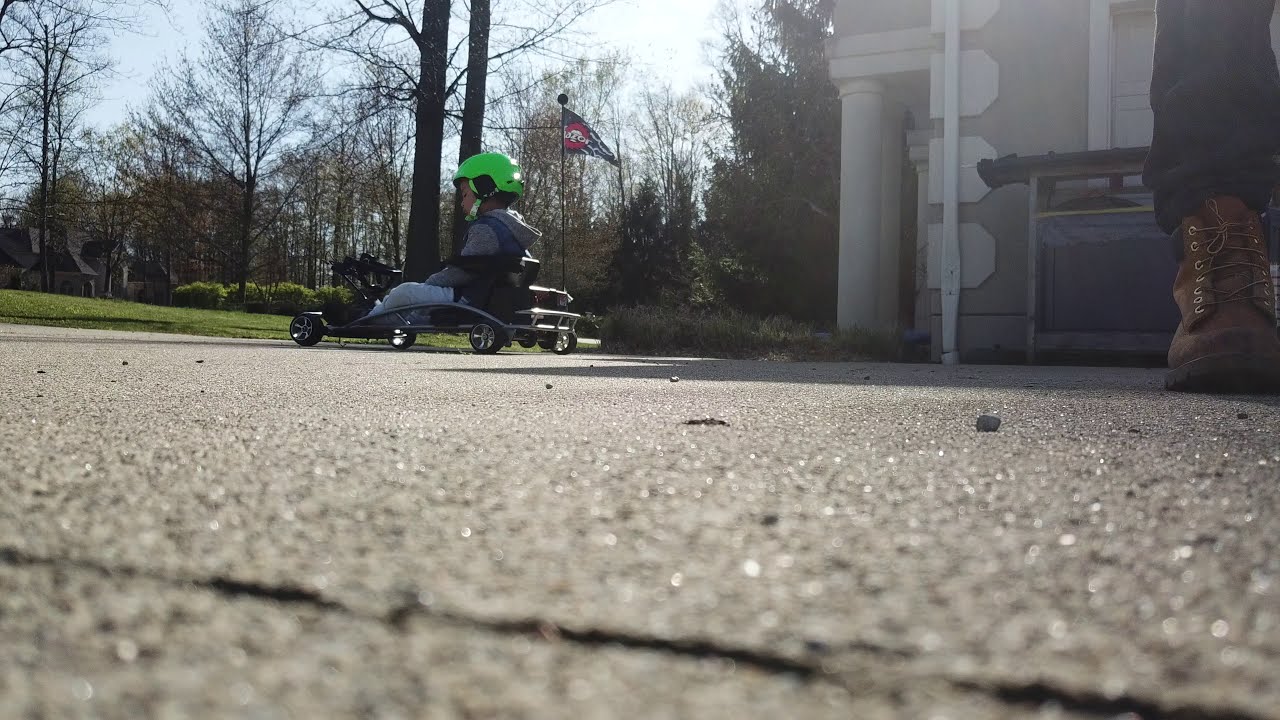In this vivid image, a young boy, around seven or eight years old, excitedly navigates a small, silver motorized go-kart on a gray concrete pavement. Donning a bright yellow-green helmet for safety, he sports a gray hoodie, possibly with a jean vest-like design, and white pants. A black and red flag flutters behind his go-kart, capturing the motion and thrill of his ride. Nearby, a parent stands, identifiable only by the brown boot and black pants visible in the top right corner of the photograph. In the background, there is a white and gray building, likely a residence, with a black and silver grill placed in front. Beyond the building, the scene extends to include a lush green grassy area with trees that are either bare or just beginning to sprout new leaves, indicating a transition in seasons, possibly spring or fall. The sky overhead is a picturesque blue with patches of white clouds, and distant brown-roofed houses add a touch of suburban tranquility. The entire scene exudes a sense of outdoor adventure and familial oversight, highlighting the boy's budding enthusiasm for his little go-kart.